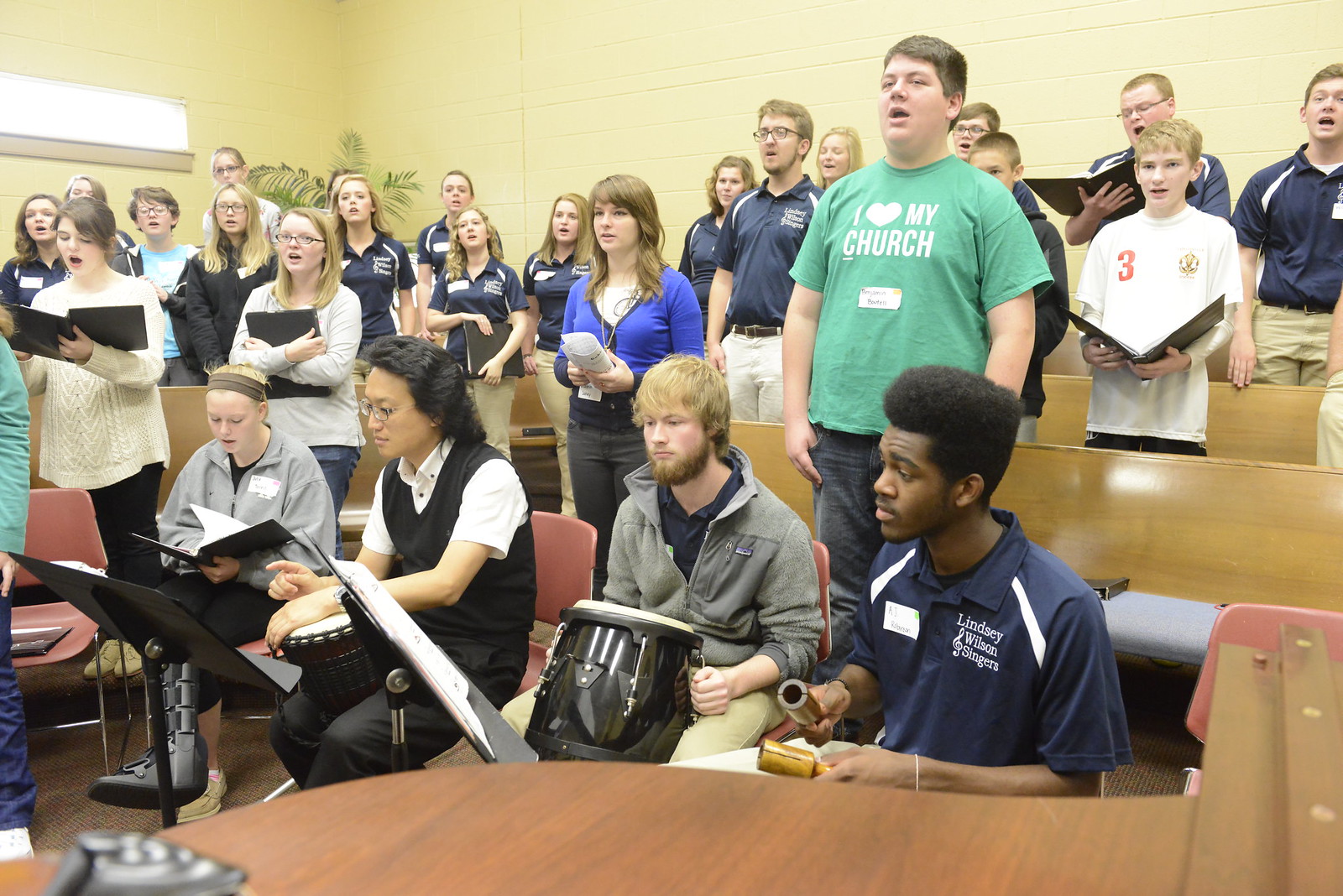The photograph captures a vibrant scene in what appears to be a music class or choir practice, possibly taking place in a church setting. The room is filled with around 25 individuals, a diverse group comprising both men and women of various racial backgrounds. Many of the people are standing, while a few are seated, creating a dynamic and lively atmosphere.

Several individuals are holding sheet music or hymn books, indicating that singing is a significant part of the activity. Some group members have their mouths open, clearly in the act of singing. The front of the room is occupied by a smaller group of about four or five people, who are seated and playing various instruments. These instruments include drums, conga drums, cymbals, tambourines, and wooden sticks being struck together, contributing to a rich, rhythmic backdrop.

Details in the image, such as a person wearing an "I Love My Church" shirt and another with a "Lindsey Wilson Singers" shirt, suggest a community or school choir practice. The color palette of the room includes shades of brown, black, white, grey, blue, green, beige, cream, and red, adding to the visual diversity of the setting. Overall, the scene is one of communal musical engagement, blending voices and instruments in a collective effort.